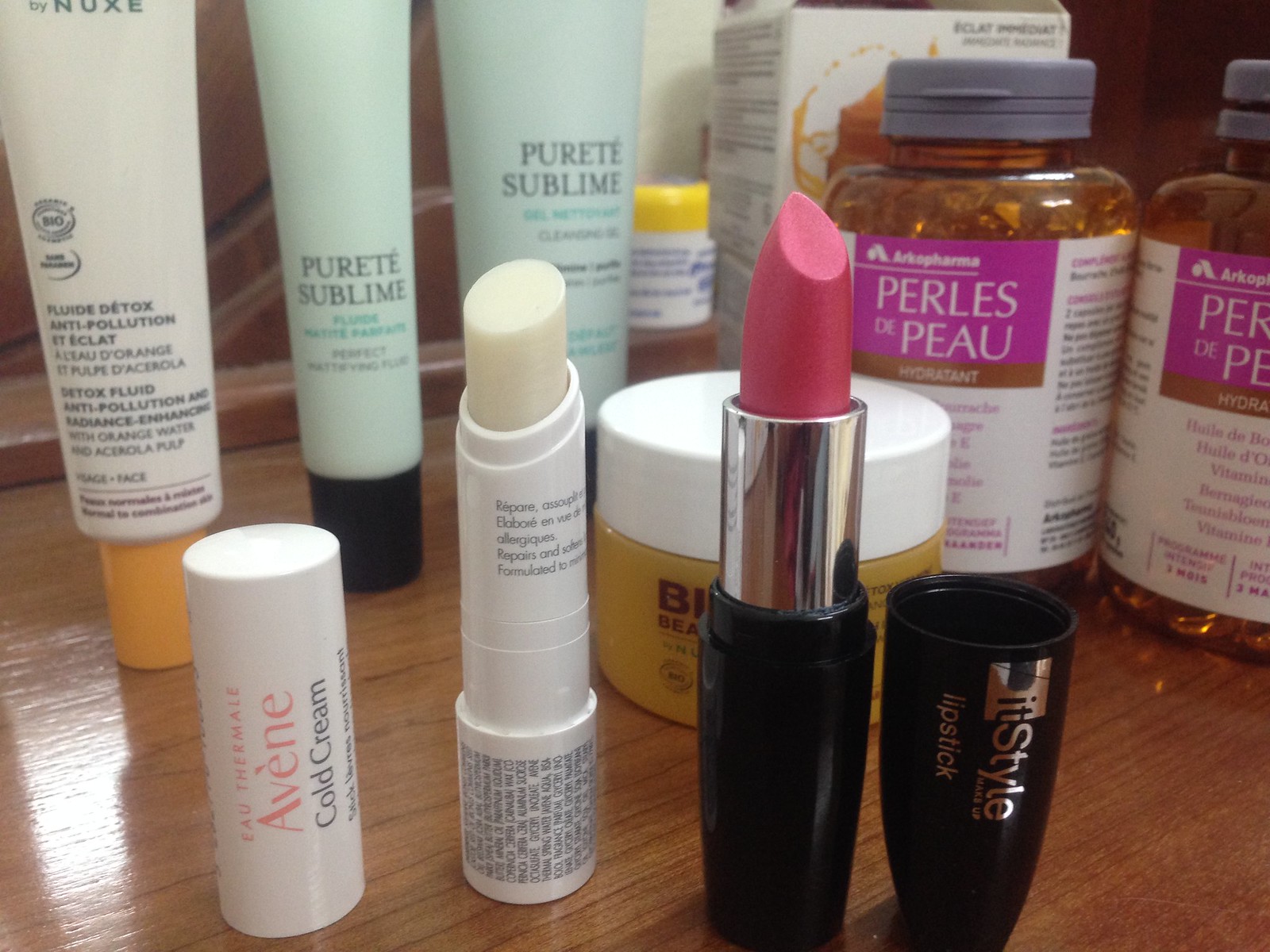In this detailed photograph, we observe an exquisite collection of beauty products meticulously arranged to provide an array of options for personal care and enhancement. Dominating the bottom right corner is a sleek black tube of lipstick, adorned with a silver trim around the inner case. The lipstick itself boasts a creamy pink hue, and the cap proudly displays the label "Style Lipstick."

Adjacent to the lipstick, on the left, is a small container of lip balm. Though the text on the side is partially in French and reads "repair," the product's specific name is not fully legible. Its cap, situated nearby at the bottom left, features the words "cold cream" in friendly, gold lettering.

Moving up to the top right of the image, a collection of bottles is visible. Among them is a hydrating lotion alongside a pill bottle labeled "Pearl Essence Deep-Hue," adding to the variety of skincare options. In the top left corner, there is a small bottle marked "Fluide Détox Anti-Pollution," which contains a cream meant to be applied to the skin for detoxification purposes.

To the right of this, a light green bottle labeled "Pure & Sublime" stands out, alongside its larger counterpart, indicating perhaps double the quantity of lotion intended for hand moisturizing. This set of personal care items collectively includes different perfumes, makeup products, and lotions, all designed to enhance beauty and provide a luxurious self-care experience.